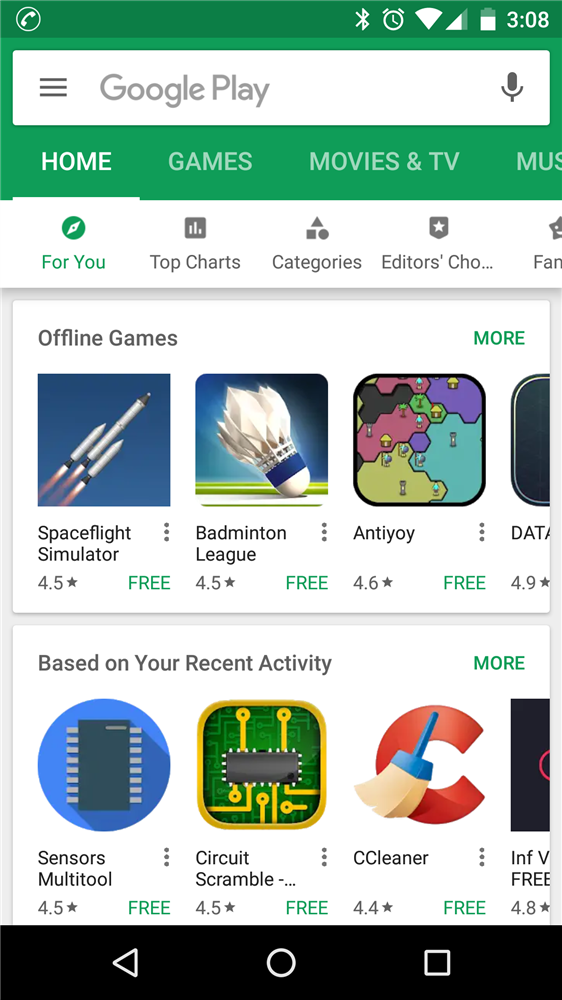The image displays a section of the Google Play Store, an online marketplace for a variety of apps, games, movies, and television shows developed for Android devices. Featured prominently are several free offline games, such as Space Flight Simulator, Badminton League, and Antioi. The selection also includes utility apps like Sensors Multitool, Circuit Scramble, and CCleaner, which offer functionalities ranging from system optimization to complex problem-solving tools. The interface presents these apps with green download buttons, indicating their "free" status. The screen is framed by a black border at the bottom, completing the layout.